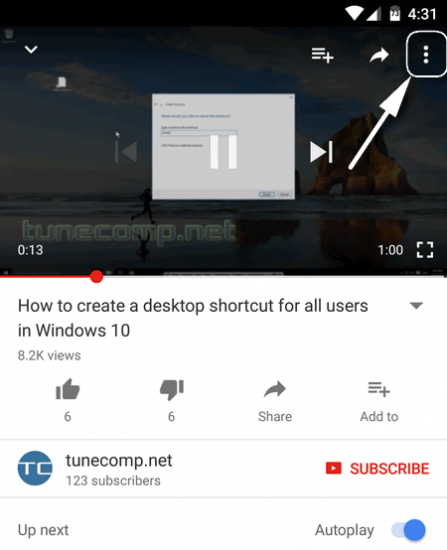This image is a screenshot displaying a YouTube video interface. The top half of the image features a black header with white textual elements. In the upper right corner, icons for Wi-Fi connectivity, cell reception, battery level, and the current time reading '4:31' are displayed. Beneath these, there are three small vertical dots outlined in gray, which have two arrows pointing towards them, indicating interaction options.

On the top left side of the header, there is a pull-down arrow. The text at the bottom of this black header indicates the source of the content, "TuneComp.net," presented in gray text.

Below the header, the title of the YouTube video is clearly shown: "How to create a desktop shortcut for all users in Windows 10," with a pull-down arrow to the right of it. Further down, the video statistics are displayed, showing 8,200 views. There are icons for six thumbs up, six thumbs down, a share option, and an 'add to' feature.

The detailed and organized layout of the interface captures the essential elements of the YouTube video information succinctly.